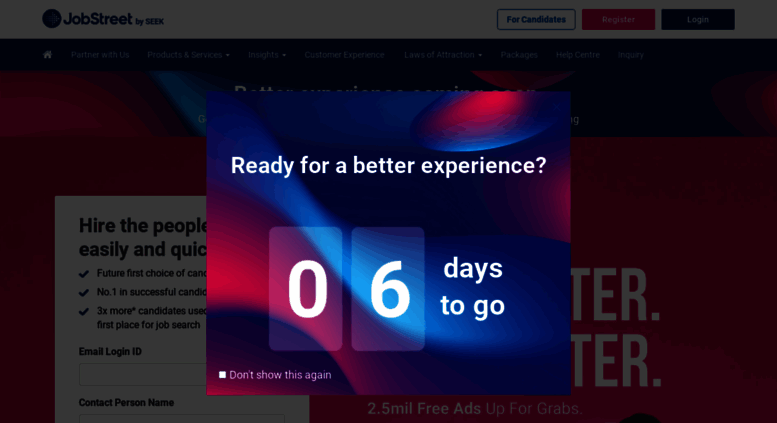On first glance, this appears to be a landing page for job seekers. In the upper left-hand corner, the webpage is branded with "JobStreet by SEEK." Positioned in the upper right-hand corner, options for candidates include "Register" and "Log In." Directly below that, a home icon is displayed alongside the options: "Partner with Us," "Products and Services," "Insights," "Customer Experience," "Laws of Attraction," "Packages," "Help Center," and "Inquiry."

A prominent pop-up box occupies the center of the screen, stating, "Ready for a better experience? Six days to go. Don't show this again," suggesting it can be minimized at the user’s discretion. This pop-up partially obscures the text behind it, which seemingly reads: "Hire the best people easily and quickly. Future first choice of candidates. Number one in successful candidate placements. Three times more candidates use us to find jobs." Additionally, the page features fields for "Email," "Login ID," "Contact Person," and space for corresponding entries. A banner also highlights, "2.5 million free ads up for grabs."